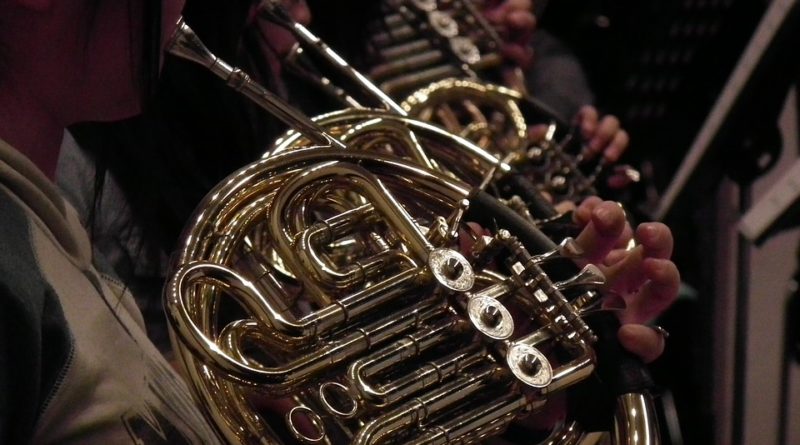This detailed photograph, set indoors, captures a close-up of three French horn players positioned next to each other, forming a small ensemble likely part of a larger orchestra or band. The focus is primarily on their brass instruments, which are gold in color and feature intricate curves and valves. In the foreground, the white fingers of the frontmost player, who is wearing a light brown and dark gray sweatshirt with a discernible letter "M," are poised on the three valves of the French horn. This player's dark hair is slightly visible as they blow into the mouthpiece. Behind them, partially obscured yet recognizable, is another player with a darker complexion, whose hands and out-of-focus face are faintly discernible. The fingers of this second player are also positioned on the valves. The composition is relatively dark, minimizing background distractions and further highlighting the instruments and the players' hands. In the bottom right corner, the white frame of a door is just visible, adding to the indoor setting's details.